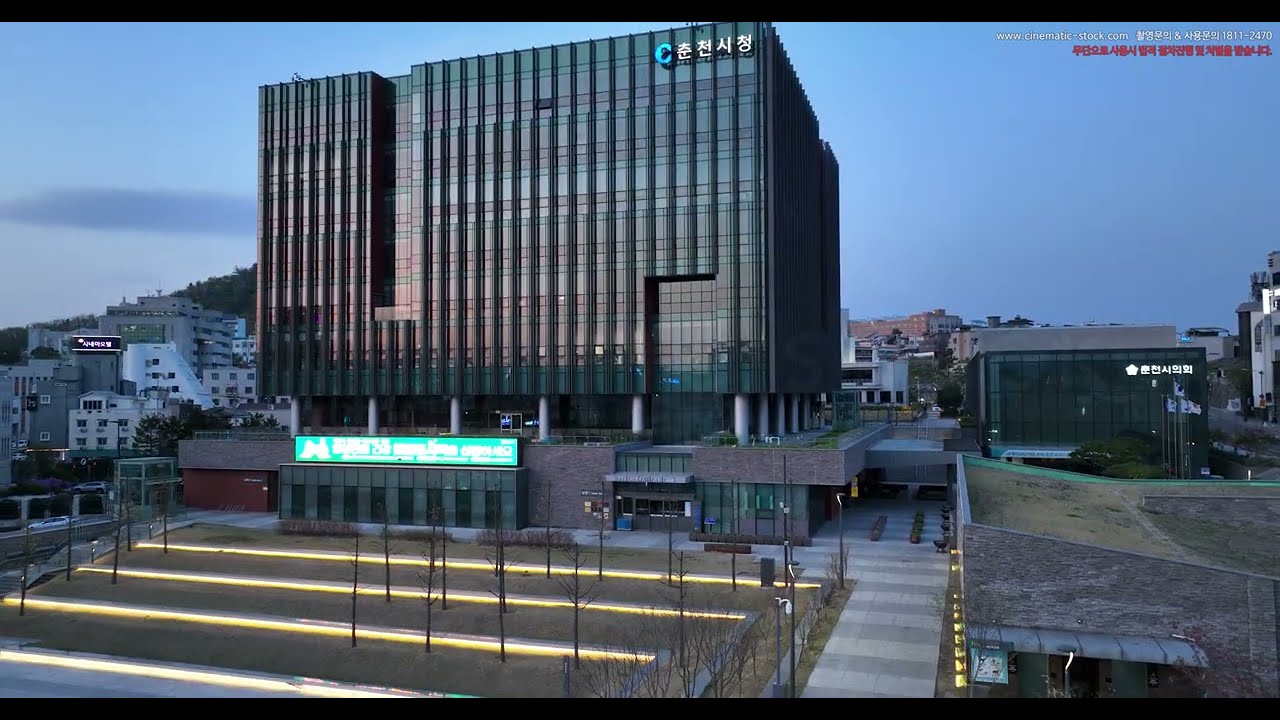A daytime photograph captures a semi-densely populated, suburban urban area situated near a hillside. The main feature, centrally positioned with a slight left tilt, is a large, seven-story office building characterized by its glass and metal façade and a distinctive Chicago-style architecture. Notably, a deep indent carves through a third of the building's structure, while the lower level, resting atop a brick or stone building, hosts various shops and a walking area. Asian symbols, predominantly Chinese characters, prominently adorn the top right corner of this silver-hued building and the adjacent smaller structure to its right. The foreground features a tiered grassy area, illuminated by ground lighting, and accented with bare trees resembling large twigs. Framing this central building are additional structures and houses, each adorned with similar Asian symbols. The sky above is a clear, vivid blue with minimal cloud cover, and the overall ambiance suggests an early evening or late afternoon setting, as light subtly hints at the onset of dusk.